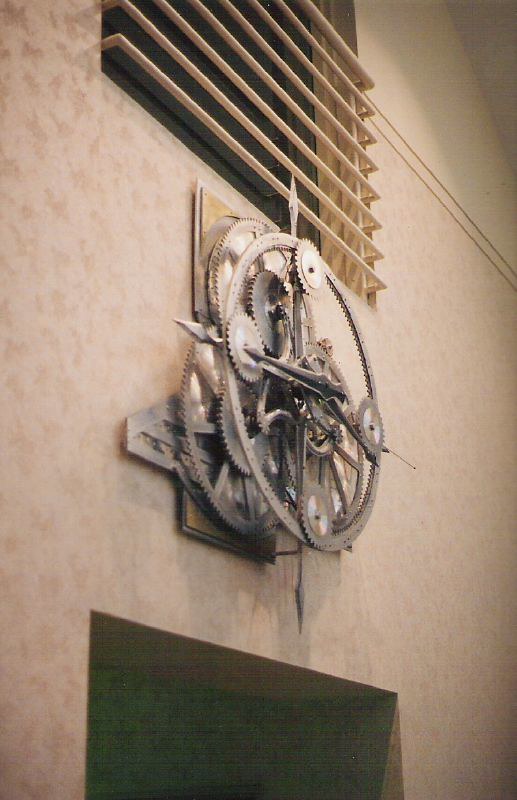This is an image of a tan wall featuring a small, barred window with eight vertical bars, also painted tan. Prominently mounted on the wall is a large, face-less mechanical clock displaying its intricate, exposed metal mechanisms. The clock's hands, made of black metal, point towards where the numbered positions would typically be found. Instead of numbers, the positions at 12, 3, 6, and 9 are marked by additional visible gears, contributing to the industrial aesthetic of the timepiece. The overall scene blends stark mechanical elements with a muted, monochromatic color scheme.